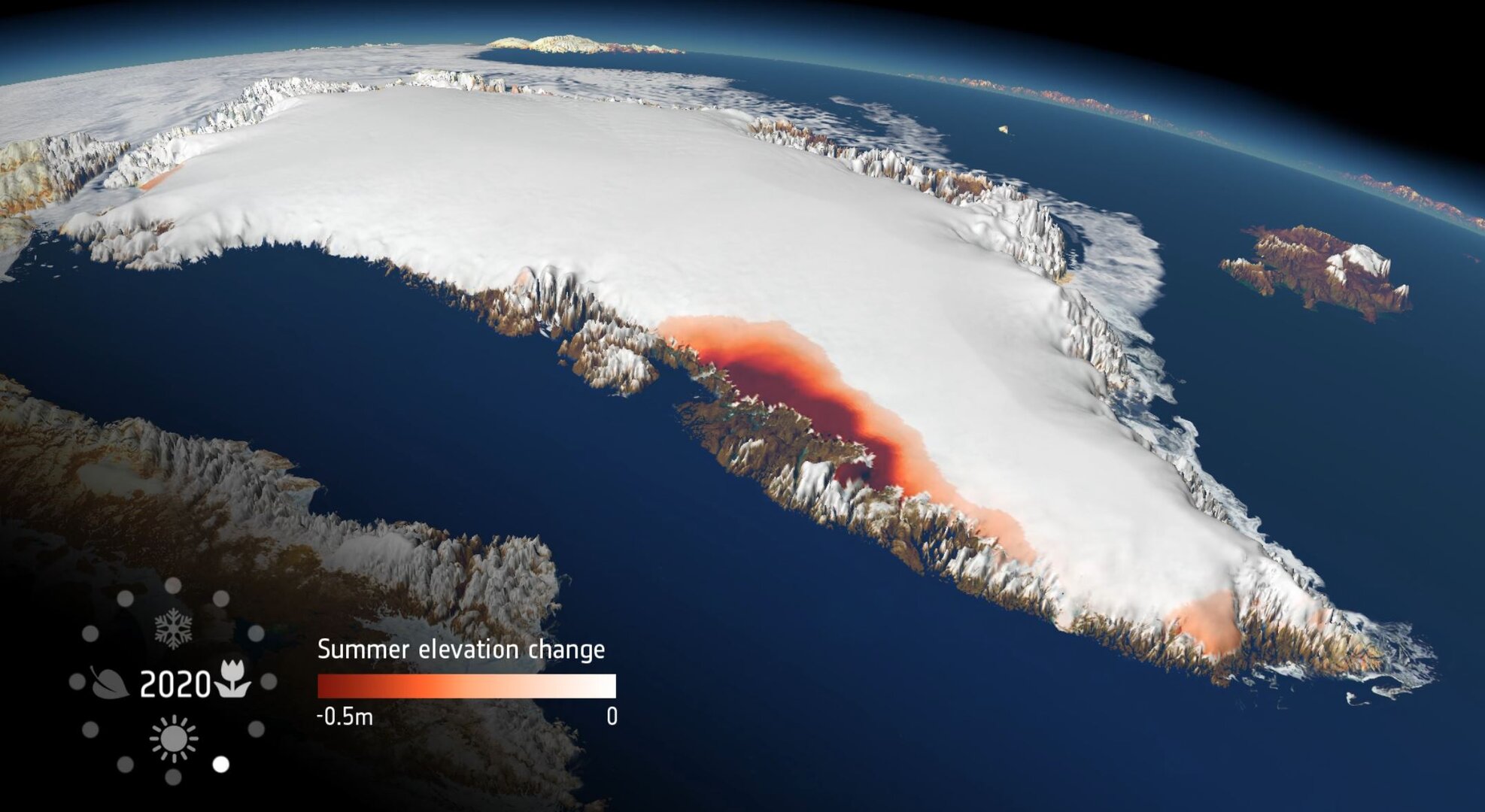The image is a digitized 3D rendering of Greenland, displaying its topography and seasonal elevation changes. Set against a backdrop of dark blue water, the landmass appears extensively covered in snow or ice, with a particularly dark red region indicating significant elevation change. The overall shape of the image is rectangular, with the top and bottom sides being twice as long as its width. In the left-hand corner of the image, a semi-transparent grey circle composed of dots contains symbols representing the four seasons: a snowflake at the top, a flower to the right, a sun at the bottom, and a leaf to the left. Inside the circle, the white text reads "2020." Adjacent to this, there's a bar that illustrates the summer elevation change, ranging from dark red (indicating -0.5 meters) to white (indicating no change). In addition to the primary landmass of Greenland, a smaller adjacent landmass is depicted in brown, further emphasizing the detailed topographical features of the region.